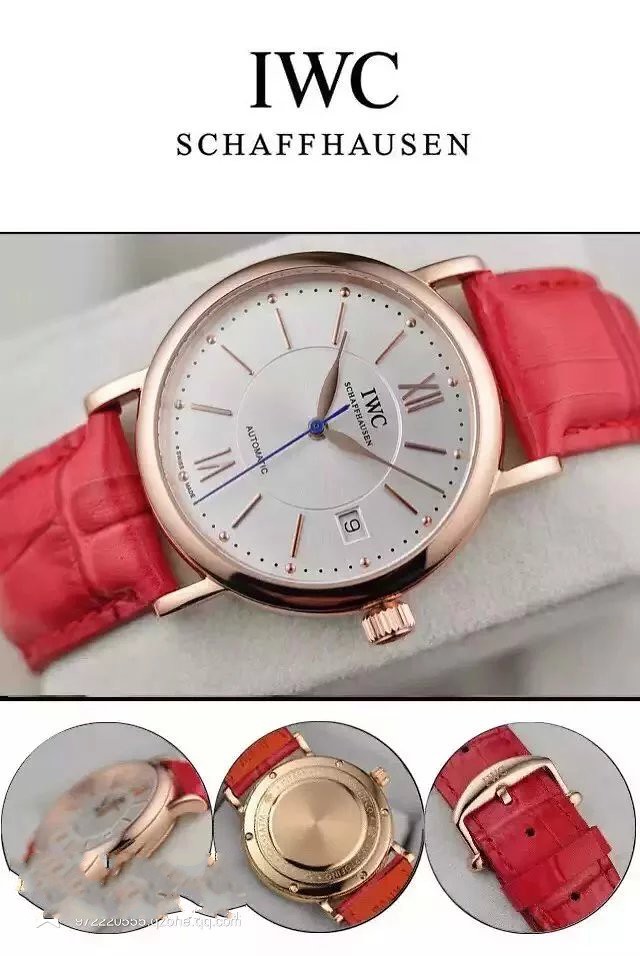This image depicts a sophisticated IWC Schaffhausen wristwatch with a reddish-pink, likely leather, band. The watch face prominently features "IWC" in a large black font, with "Schaffhausen" in smaller black capitals underneath it, positioned below the 12 o'clock marker. The watch has a gold casing, a white dial, and distinct gold Roman Numerals for 12 and 6, while the remaining hour markers are single vertical lines. The hour and minute hands are crafted in gold, contrasting with a striking blue second hand. On the lower half of the face, just above the 6 o'clock position, the word "Automatic" is printed. Below the main display are three smaller circular images showcasing different angles of the watch: a detailed side view (though blurry), a rear view highlighting the back of the watch, and a close-up of the band and its gold clasp. The advertisement provides a comprehensive view of the elegantly designed watch and its components.